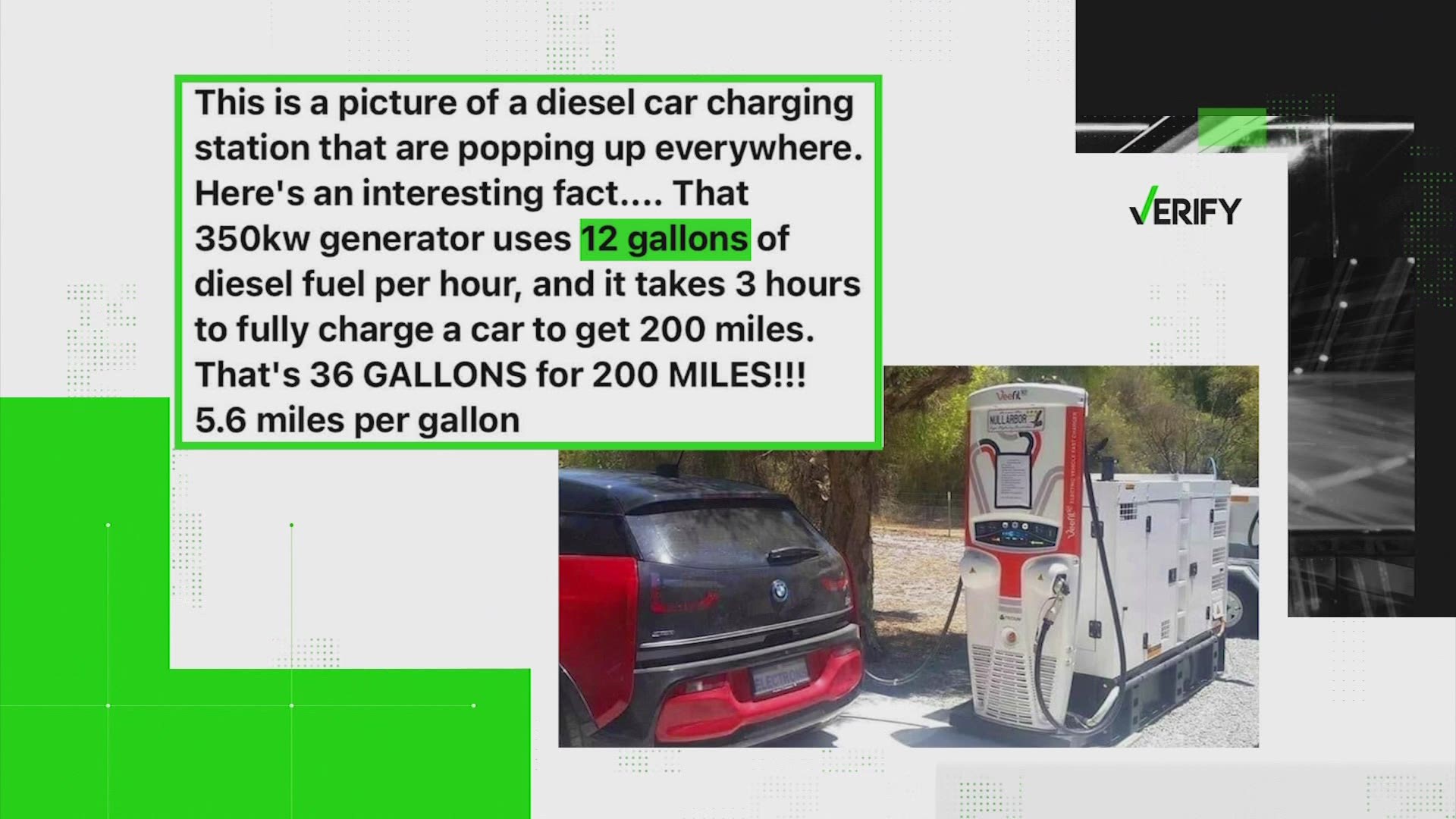This detailed image appears to be a rectangular PowerPoint slide, approximately five to six inches wide and three inches high, with a light gray background. In the bottom right corner, there's a photograph of a black and red SUV connected to a small white charging station resembling a gas pump, featuring black exhaust pipes, controls, vents, and a red accent. This diesel generator, highlighted with a vibrant green, uses 12 gallons of diesel fuel per hour and takes three hours to fully charge the car for a range of 200 miles, consuming 36 gallons for those 200 miles, equating to 5.6 miles per gallon. The ground around the station is a mix of short-cut grass, gray gravel, and sparse brown trees with patches of green leaves, giving the impression of a dry, almost desert-like environment. The upper left corner contains a light bright green rectangular outline with a black text box inside, stating: "This is a picture of a diesel car charging station that are popping up everywhere. Here's an interesting fact: that 350 kW generator uses 12 gallons of diesel fuel per hour and it takes three hours to fully charge a car to get 200 miles. That's 36 gallons for 200 miles, 5.6 miles per gallon." Additional geometric shapes, including vibrant green and dark gray L-shaped blocks, populate the image, along with miscellaneous green squares and white squares scattered throughout. A black box with white lines sits on the right, marked with the word "verify," and a partially visible platform in the upper right corner adds to the intricate layout of this visually engaging, seemingly critical depiction.